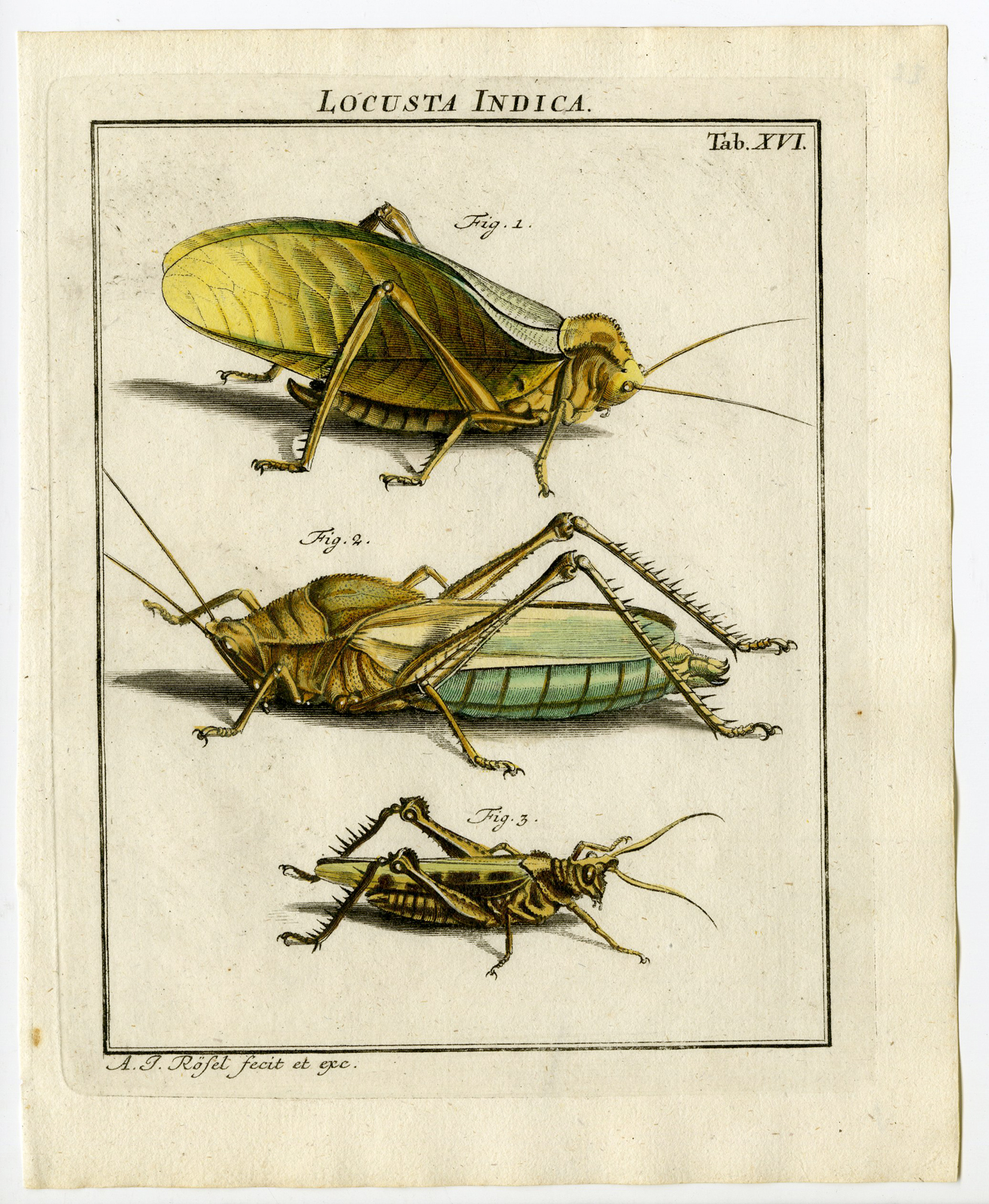This image features a detailed, artistic diagram illustrating three distinct stages or variations of the locust species Locusta Indica, sketched by the artist A.J. Raphael (Fessit Exe), set against a white background. At the very top, the diagram introduces the subject with its Latin name. The first figure, positioned at the top, depicts a large locust facing right, characterized by prominent vertical wings and lengthy antennae. The middle figure, facing left, displays a locust with large, spiky legs and slightly flatter wings, giving it a more cricket-like appearance. The final figure at the bottom presents a much smaller locust, with wings lying flat on its back, facing right, and detailed with green coloring, spiky legs, and small eyes. This comprehensive visual captures various physical attributes and stages of the locust, offering an insightful view into the species' morphology.